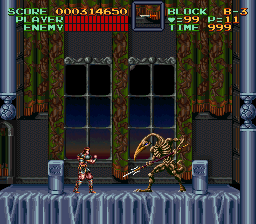This color screenshot from a video game, potentially resembling Castlevania from the Nintendo or Sega era, features a dynamic battle scene. The game's status bar, located at the top left corner of the image, displays various metrics in green text: "Score: 31,4650," indicating the accumulated points; "Player" and "Enemy" health bars, with both entities missing one bar of health. The selected weapon is shown in a box at the center of the top bar. To the right, additional information in green reads "Block B3," "Heart = 99," "P = 11," and a timer counting down from 999 seconds. In the main action scene, two characters are locked in combat: one, outfitted in colonial or Roman-like armor with a shield, and the other appearing as a skeletal dinosaur wielding a sword.